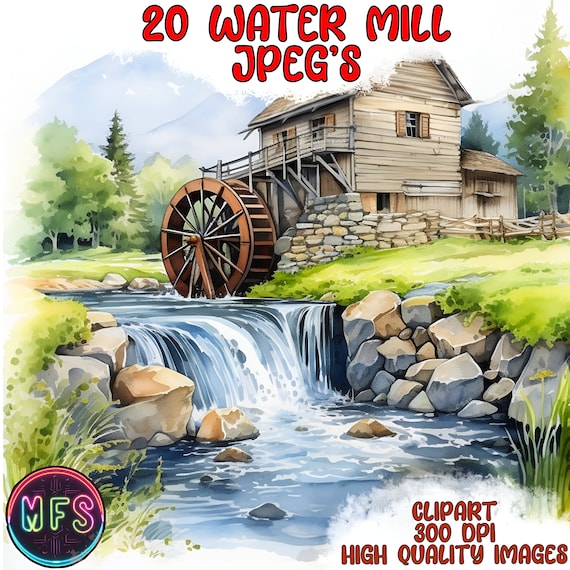This detailed color illustration depicts an old wooden water mill with an unfinished wood-cladded siding, brown shutters, and a peaked brown roof. The mill features a large wooden water wheel positioned prominently in front, next to the stream. The stream in the foreground showcases a blue and white waterfall, with the water turning white as it cascades down. On either side of the creek are imposing stone walls made of big boulders, bordered by patches of grass. A wooden post fence is visible to the right of the mill, while a line of trees and a mountain are set in the distant background.

Red text at the top of the image reads "20 Watermill JPEGs," and in the lower right corner, there is text stating "Clipart 300 DPI High Quality Images." Additionally, a circle on the lower left corner contains the letters "MFS."